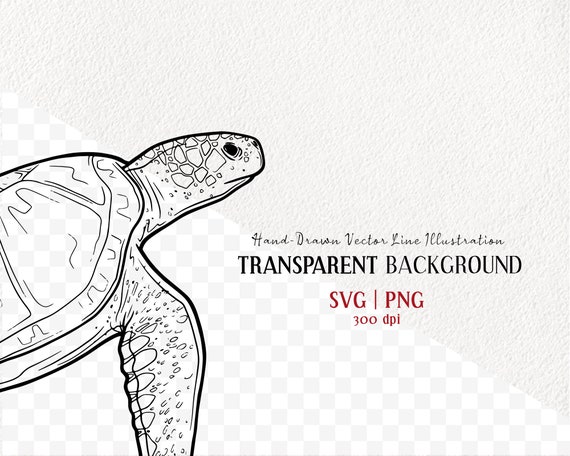The image is a detailed black-and-white illustration of a sea turtle, captured in a hand-drawn vector line style. The turtle, facing right, showcases intricate details such as his eye, the mottling on his skin, and the distinct sections of his shell. Surrounding the turtle's face are small squares, adding texture to the illustration. The background is split diagonally; the top half features a gray, textured pattern, while the bottom half displays a muted gray and white checkerboard design. Prominently featured text on the image reads "Hand-drawn vector line illustration" and "Transparent background" in bold letters, with "SVG/PNG 300 DPI" written in red below. This image appears to serve as an advertisement or educational resource, possibly for a book or guide on creating similar light, transparent illustrations.